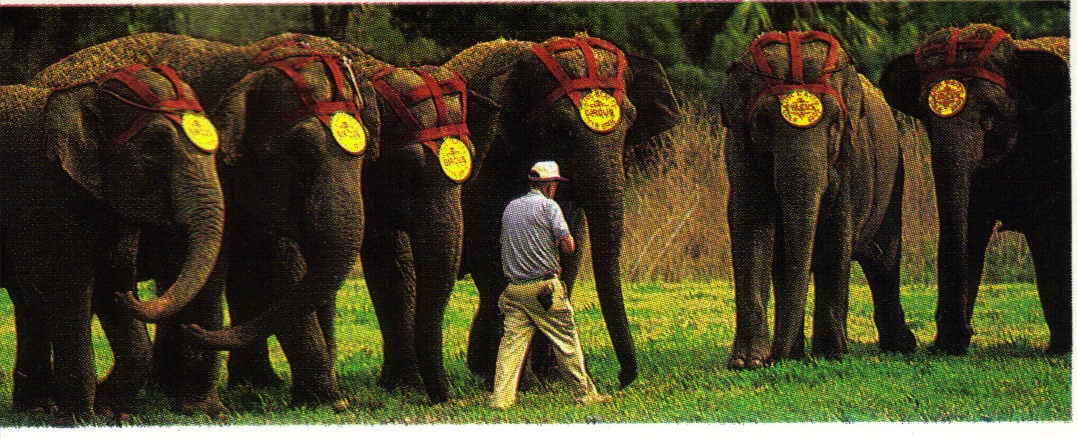In this outdoor nature scene, a grassy lawn is the central focus, where six large, dark grayish-brown female elephants are standing, all looking toward the camera. Each elephant is adorned with a distinctive red headdress featuring a prominent gold disc at the center, although the specific logo on the discs remains indistinguishable. The elephants are arranged in a row with a small gap between them, four on one side and two on the other. In front of them, a man is captured mid-step, facing the elephants. He is dressed in a light blue short-sleeved shirt, beige khaki pants, and a white hat, with an unidentified item sticking out of his back pocket. The background of the image features tall yellow grass in front of a dense row of trees with dark green leaves, completing this vivid, rectangular-shaped photograph.